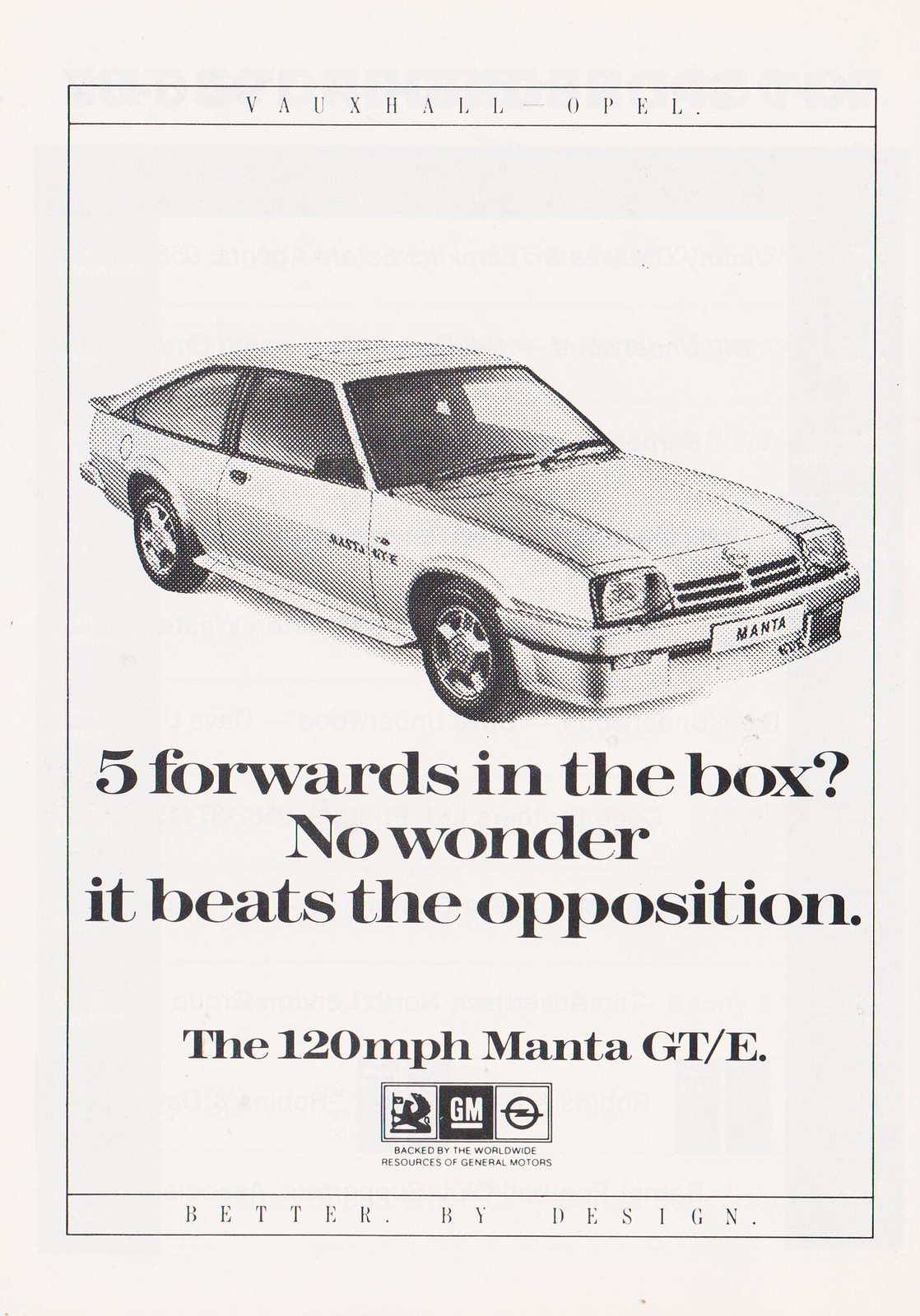This black-and-white print advertisement from Vauxhall-Opel features a hand-drawn style image of a two-door Manta GT/E car, viewed from an angle where the front right headlight is closest to the viewer. The car is illustrated against a white background with prominent text below it. At the top of the ad, "Vauxhall-Opel" is displayed in black writing. Directly below the car’s image, a plate with the name "Manta" is visible. The advertisement text includes the phrase, "Five forwards in the box? No wonder it beats the opposition." It also states, "The 120 mile per hour Manta GT/E." Beneath this, logos are shown, including that of General Motors (GM) among others, indicating the car's backing by GM's worldwide resources. The slogan at the bottom reads, "Better by Design." The overall composition suggests it’s a historical advertisement reflecting the car's performance and design attributes.